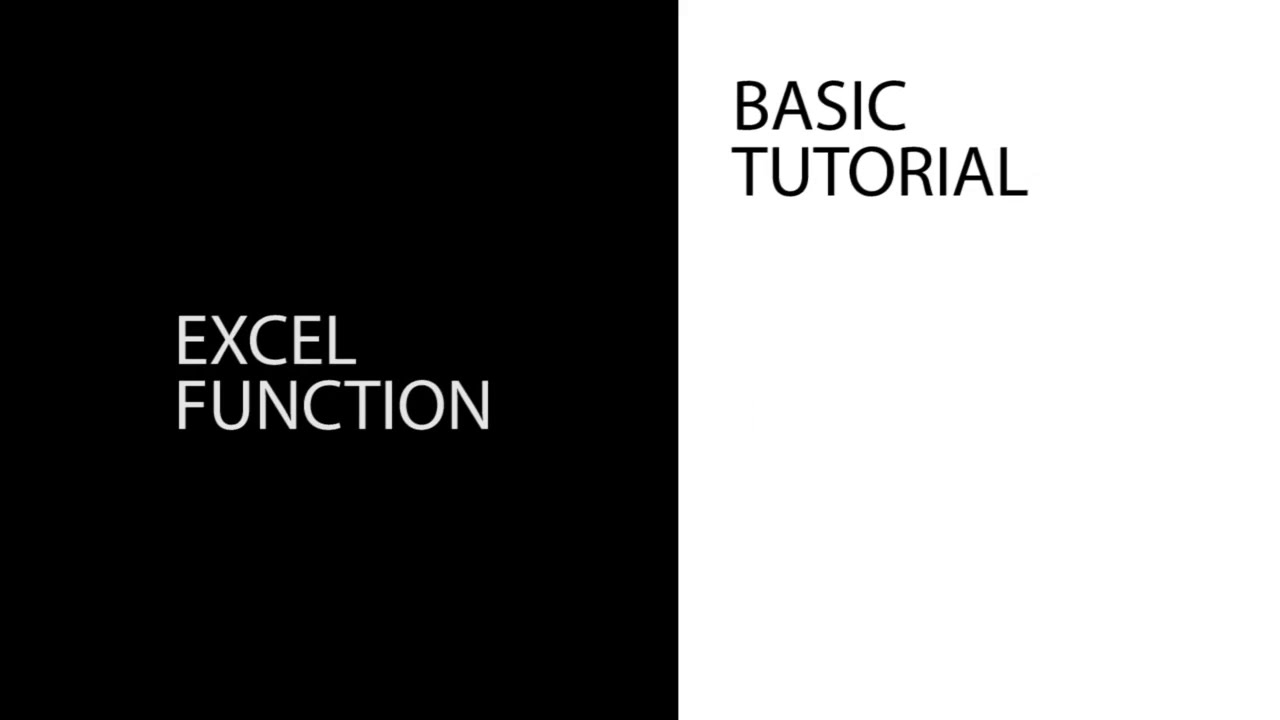The image depicts a minimalist design split into two sections, creating a stark contrast. On the left-hand side, there's a prominent black square with the words "Excel" and "Function" in all capital letters, centered in the middle in white font. The word "Excel" is positioned directly above "Function," creating a vertical alignment. On the right-hand side of the image, against a blank white background, the phrase "Basic Tutorial" appears in black text. The words "Basic" and "Tutorial" are stacked on two separate lines near the top left corner of the white area. The overall layout is clean, with a basic font and a clear division between the black and white sections, suggesting a simple and straightforward tutorial interface.